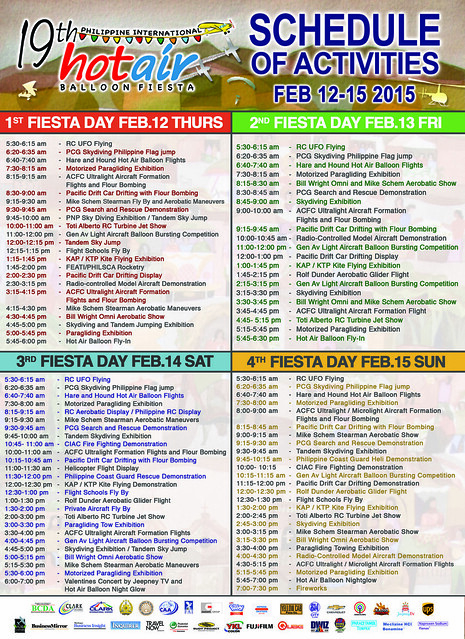This is a detailed poster for the 19th Philippine International Hot Air Balloon Fiesta, held from February 12th to 15th, 2015. The poster is visually striking with a colorful design and a background featuring houses. The event title "Hot Air Balloon Fiesta" is prominently displayed with "Hot" in red and "Air" in blue. Each of the four days is color-coded and listed with the corresponding date and day of the week: 

- The 1st Fiesta Day, February 12th (Thursday), in red.
- The 2nd Fiesta Day, February 13th (Friday), in green.
- The 3rd Fiesta Day, February 14th (Saturday), in blue.
- The 4th Fiesta Day, February 15th (Sunday), in yellow.

Each day brims with around two dozen activities, including notable events like the RC UFO flying sessions starting each morning and a skydiving exhibition at 8:45 a.m. on the second day. At the bottom of the poster, there is an array of logos representing various sponsors who support the event. The schedule is designed like a menu, making it easy to navigate through the numerous activities planned for this festive occasion.